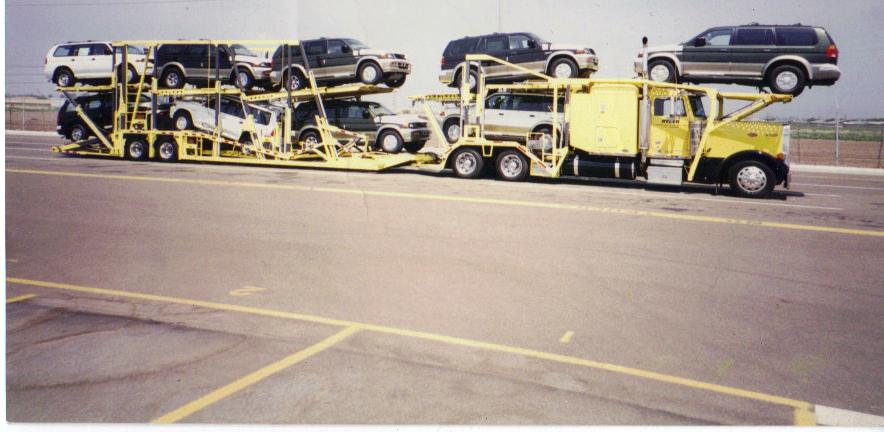The image is a grainy, color photograph from the early to mid-2000s, featuring a light yellow 16-wheeler car transporter parked in an asphalt area lined with yellow parking spaces. The foreground shows numbered parking spaces, indicating a structured parking lot. The transporter has a distinctive frame over its cab and is carrying a total of nine large SUVs, likely of the same make and model. The SUVs are arranged with one perched directly above the cab and another right behind it, facing backwards, while the remaining vehicles are oriented forwards. The load includes three white SUVs and several navy blue ones. Beyond the giant transporter truck, there’s a chain-link fence with a field in the background, potentially suggesting a rural environment or possibly a dealership lot. The overall quality of the photo is not high, with washed-out colors and poor focus, indicative of its age.